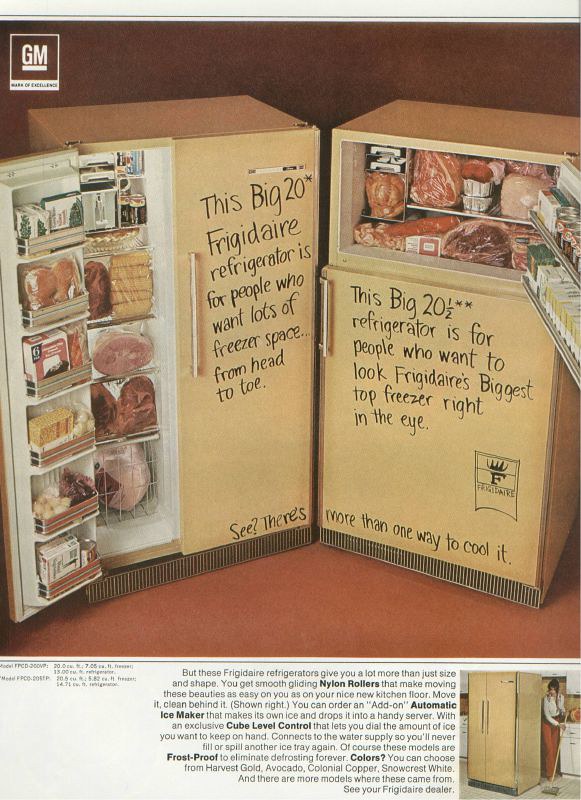This vintage advertisement from an old magazine features two Harvest Gold Frigidaire refrigerators by GM General Motors. The ad, set against a dark background with a rusty orange floor, showcases the models side-by-side. On the left, a refrigerator with French doors has its left-hand freezer door open, revealing an impressive stock of meats, corn on the cob, and other vegetables. Written in black font on this appliance, it states, "This big 20 Frigidaire refrigerator is for people who want lots of freezer space from head to toe." This message continues onto the adjacent refrigerator, which features a top freezer and bottom refrigerator design. It boasts, "This big 20 and a half refrigerator is for people who want to look Frigidaire's biggest top freezer right in the eye." The right-hand refrigerator also has its top freezer door open, similarly packed with various meats and foods. 

At the bottom of the ad, there's additional text highlighting the features of these refrigerators, such as smooth gliding nylon rollers for easy movement, an optional automatic ice maker with exclusive cube level control, and frost-proof technology to eliminate defrosting. The advertisement also offers a glimpse of one of these refrigerators in a kitchen setting, with a woman cleaning the floor behind it. The ad concludes with a note about the available color options—Harvest Gold, Avocado, Colonial Copper, and Snowcrest White—and encourages readers to visit their Frigidaire dealer.